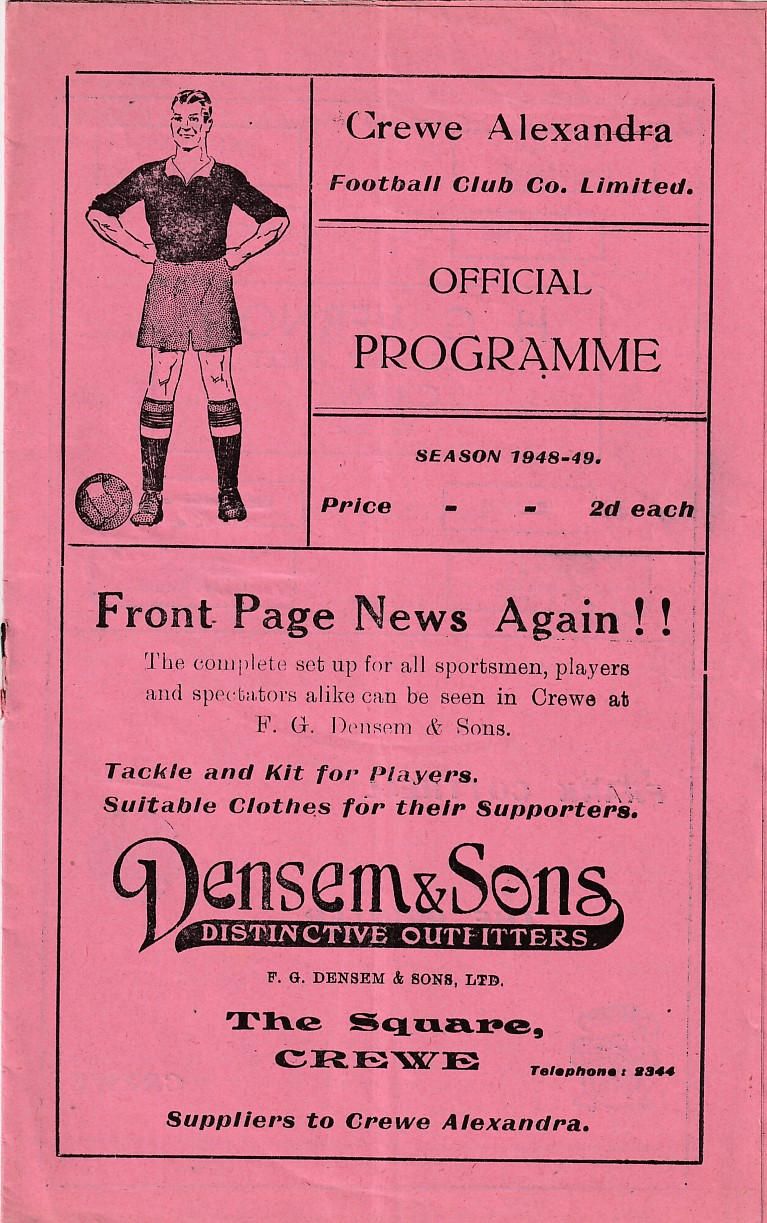This photograph features a vintage official program from the Crew Alexandra Football Club Company Limited, dating back to the 1948-1949 season. The rectangular program is predominantly pink with all text printed in black ink. Staple-bound, the cover prominently displays the club's name and its designation as an "Official Program," priced at 2D each. 

On the upper left side of the program, there’s an illustration of a soccer player. The player is depicted wearing a black jersey, gray shorts, black socks, and black shoes, standing with hands bent at the elbows and placed on his hips, with a soccer ball positioned near his right foot.

To the right of the illustration, the text reads:
- "Crew Alexandra Football Club Company Limited"
- "Official Program"
- "Season 1948 to 1949"
- "Price 2D each."

Further down, the program announces in bold, "Front Page News again!!" and goes on to promote:
"The complete setup for all sportsmen, players, and spectators alike can be seen in Crew at FG Denson and Sons. Tackle and kit for players, suitable clothes for their supporters." Below this promotional content, the logo and contact details of FG Denson and Sons Distinctive Outfitters are provided, including an address at The Square, Crew, and Telephone 2344, with a final note specifying them as "Suppliers to Crew Alexandra."